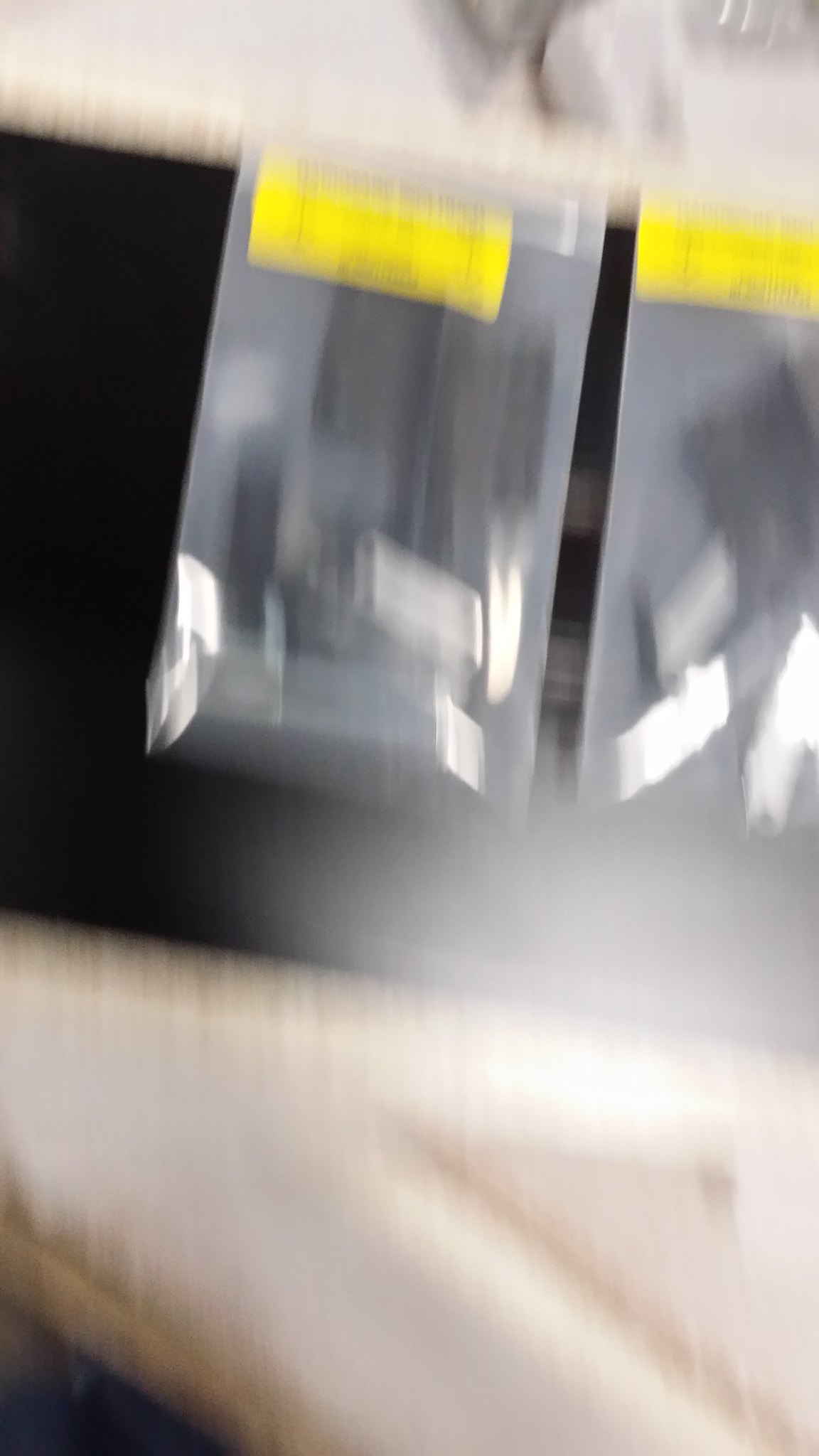This is a blurry, out-of-focus photograph depicting two clear, see-through plastic bags hanging from a beige bar. Each bag bears a yellow sticker at the top and contains indistinguishable silver and black objects, possibly mechanical parts or pieces of metal for assembling furniture. Both bags are resting on a black object positioned on an off-white surface with a marble-like texture. There is a noticeable light flare reflecting off the bags, likely from natural light coming from the right side, suggesting a nearby window. In the foreground, an additional marble-textured counter and a piece of paper are visible, while to the left, there's a shadowy area which seems to indicate another set of black drawers or surfaces. The overall composition and details are difficult to discern due to the image's low quality.